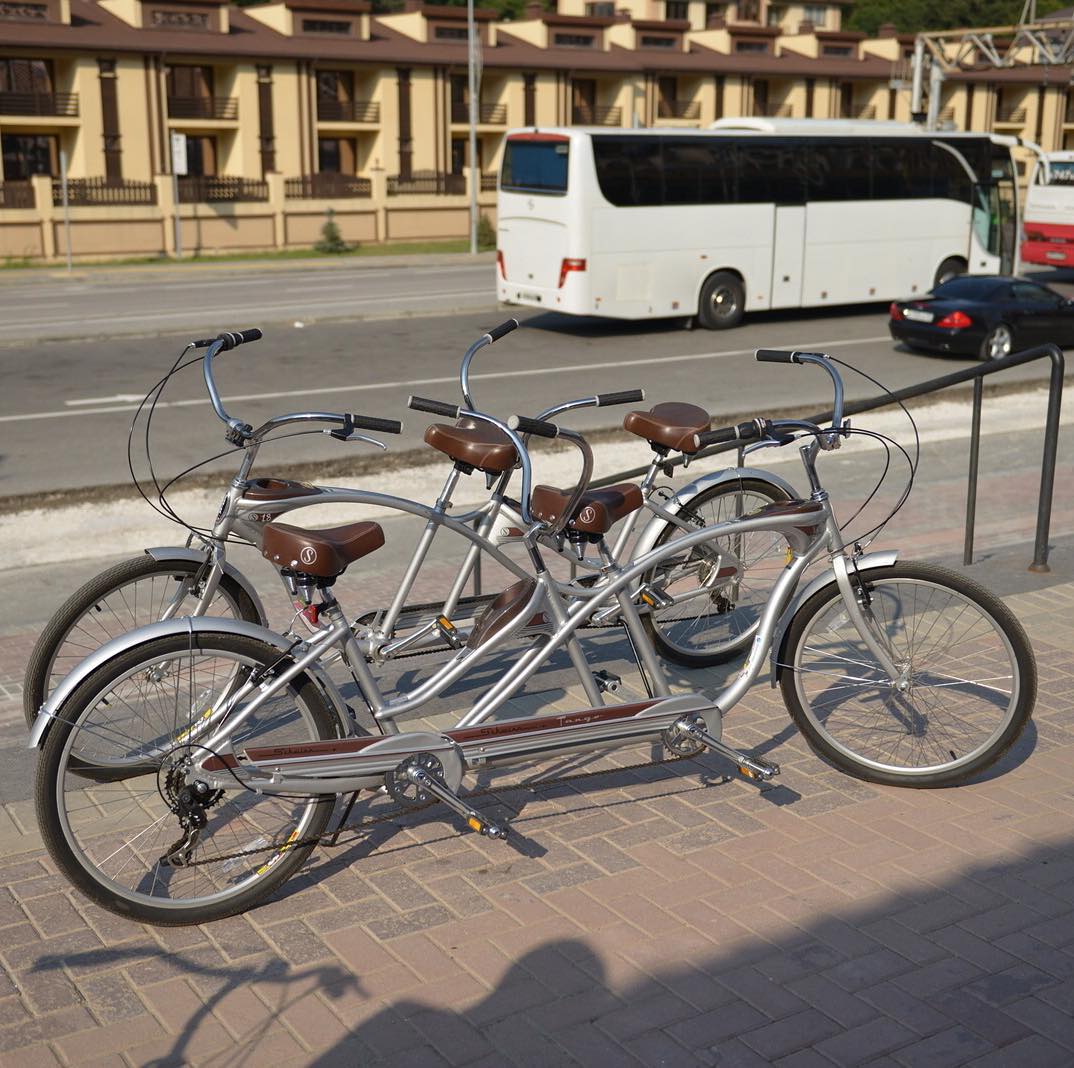In this vibrant outdoor city scene, a brick walkway leads to a set of stairs with a black metal railing, casting stark shadows under the bright sun. Dominating the foreground are two antique-looking tandem bicycles with silver frames, tall black handlebars, and brown leather seats, one facing left and the other right. The photographer's shadow, along with their bicycle's handlebars, is visible in the lower part of the image, hinting at their proximity to the intriguing vintage bikes. Beyond this setup, a busy road runs horizontally through the scene. On this road, a sleek small black car and a larger white tour bus travel from left to right. The backdrop features a long tan building with sunlit brown roofs and detailed fencing of tan stone and brown metal that might be residential apartments or row housing. The complexity and layers of this urban snapshot, from the brick pavement to the bicyclist's presence and orderly yet lively streetscape, create a rich, detailed view of a bustling city life.